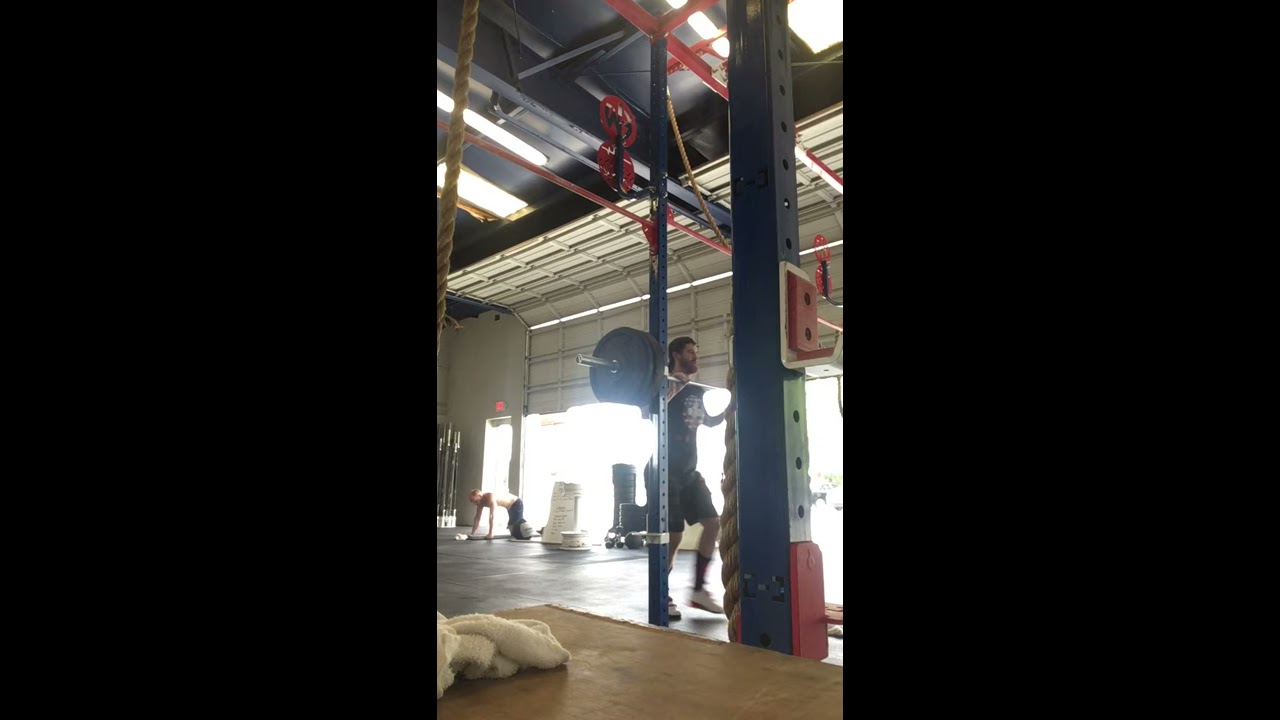The image depicts a well-lit makeshift gym within a garage, illuminated by both natural light from an open garage door and overhead artificial lighting. Two men are engaged in their workout routines. In the foreground, a man is seen holding a heavily weighted barbell, poised to begin an exercise, possibly squats. He’s standing upright, preparing for his lift. Behind him, another man is shirtless and positioned on his hands and knees, suggesting he is about to start push-ups. The gym area is scattered with weights, and a towel is casually placed on top of a wooden box at the front of the image. The scene is characterized by a mix of black, white, red, and brown colors, providing a vivid and detailed snapshot of this impromptu gym setup. Overall, the setting evokes a bright and energetic atmosphere conducive to working out.